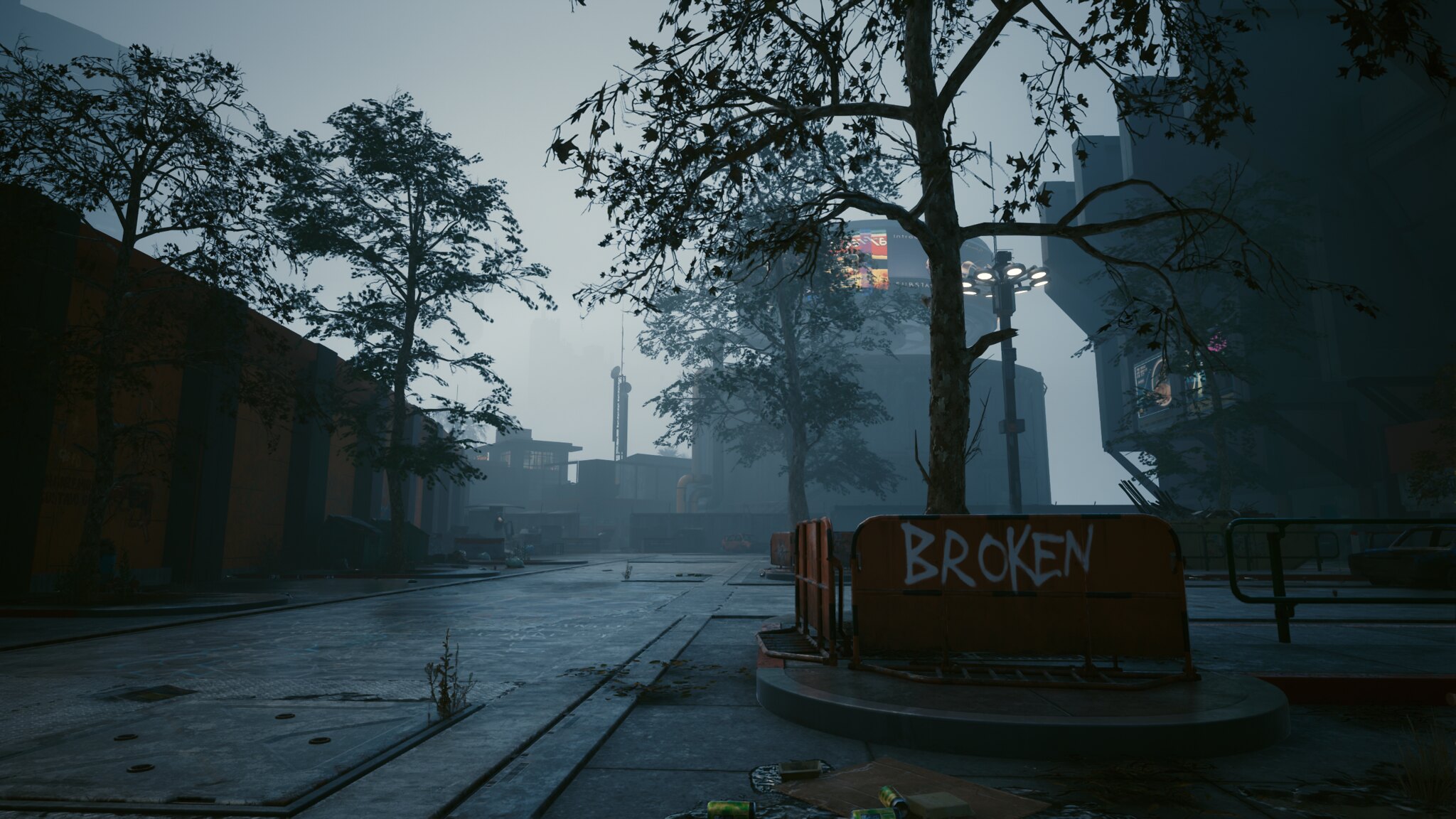In this photograph taken during twilight, a foggy, deserted city street extends into the distance, enveloped in dusky darkness. The sky is a murky gray, intensifying the eerie atmosphere. Prominently, on the right-hand side, a tall, young tree with sparse leaves stands surrounded by large, red metal barriers adorned with white graffiti that spells "BROKEN." This area could serve to block traffic or as bike racks. Directly behind this tree, a towering city building rises, featuring a conspicuous lit billboard displaying indistinguishable red and yellow colors. Adjacent to this, a peculiar architectural structure looms with a round base and top, highlighted against the foggy backdrop. 

To the upper right, another noteworthy building features a concrete facade with four columns and an ornamental rooftop, possibly hinting at its use as a museum or similar establishment. The street itself is paved with gray bricks, punctuated by manhole covers and repair panels, and lined with additional planted trees. On the left side of the street, there is a single-story brick structure with evenly spaced, orange warehouse-style doors. Above it, a low, solid stone fence extends parallel to the sidewalk, ultimately leading to an unusually designed street pole crowned with a circle of white lights. This configuration casts a dim, uniform illumination, enhancing the overall somber and mysterious ambiance of the scene.